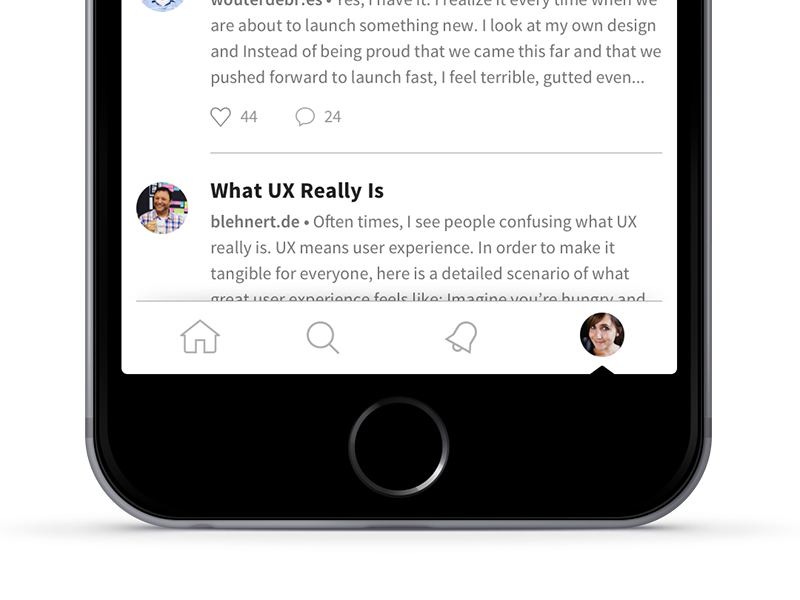The image showcases a black smartphone against a white background, positioned to display the lower half of the device. The phone screen reveals a partially visible conversation, focusing on an individual's reaction to a launch announcement. Although the top portion of the message is obscured, the legible text expresses mixed emotions: "something something are about to launch something new, I look at my own design and instead of being proud that we came this far and that we pushed forward to launch fast, I feel terrible, gutted even." This candid sentiment is acknowledged with 44 likes and approximately 24 comments. 

Beneath this text, there's a visible section of an article or post titled "What UX Really Is," attributed to Blairnerd.de. The text reads, "often times I see people confusing what UX really is, UX means user experience in order to make it tangible for everyone, here is a detailed scenario of what," with the remaining portion cut off. The image captures the essence of reflecting on the nuances of user experience design and indicates an intriguing, albeit incomplete, glimpse into a professional discourse on UX.